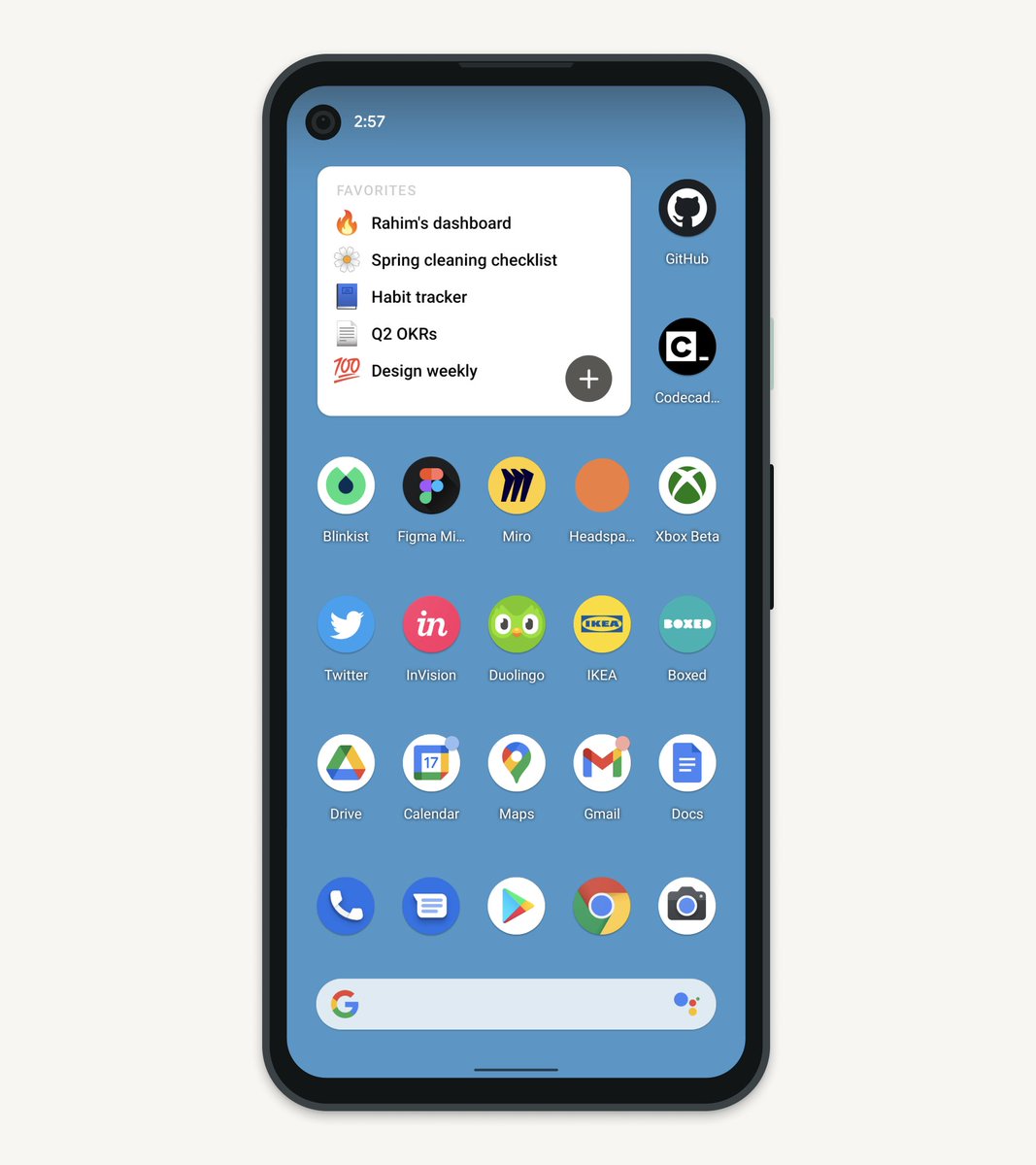In this image, we see an Android mobile device with its front-facing selfie camera positioned in the top-left corner of the device. The home screen is displayed prominently, showcasing a variety of apps arranged in a grid format. Among the visible apps are GitHub, Codecademy, Blinkist, Figma, Miro, Xspace, Xbox Beta, Twitter, InVision, Chrome, Google Play Store, Google Mobile app, Camera, Gmail, Maps, Calendar, Drive, Docs, Boxed, and Ikea. A navigation bar is evident at the bottom of the screen, providing access to essential functions such as back, home, and recent apps. The overall sleek design and organization give the device a modern and user-friendly appearance.